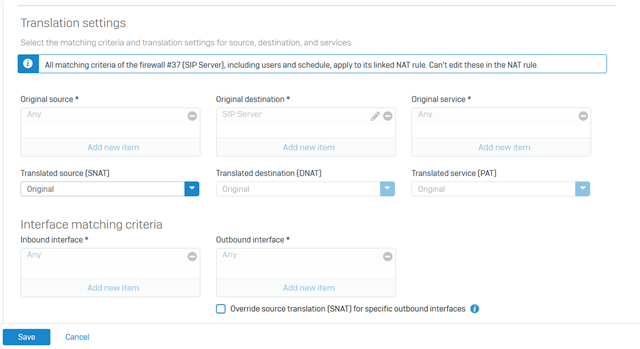This image displays the configuration interface of a firewall setup screen, where users can define various translation settings and matching criteria for both source and destination parameters. The firewall manages the translation settings for source, destination, and services, applying all matching criteria to a specific NAT rule linked to the number 37 SIP server. Notably, users cannot edit the matching criteria directly in the NAT rule.

Detailed fields include:
- Original Source and Translated Source
- Original Destination and Translated Destination
- Original Services and Translated Services
- Outbound Service
- Interface and Inbound Interface
- Override Source Translation
- Specific outbound interfaces for SNAP

Options to save or cancel the settings are prominently displayed, ensuring that all adjustments are securely applied or reverted.